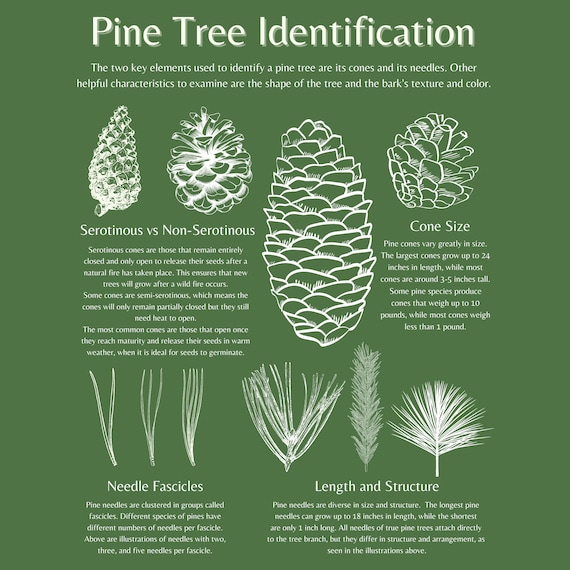The image is an identification reference guide for pine trees, titled "Pine Tree Identification," displayed in white text on a sage green background. At the top, a two-line introductory text explains that the key elements for identifying pine trees are their cones and needles, with additional characteristics such as the tree's shape and bark texture being helpful.

The central feature of the guide is a large vertically-oriented sketch of a pine cone with text and images arranged around it. To the left, two smaller images illustrate the difference between Serotoninous and Non-Serotoninous cones, explaining that serotoninous cones remain closed until exposed to fire, allowing post-wildfire germination, whereas non-serotoninous cones open at maturity to release seeds in warm weather.

On the right, another small image labeled "Cone Size" discusses the range in size of pine cones, noting that the largest can grow up to 24 inches and weigh up to 10 pounds, though most are 3-5 inches long and weigh less than one pound.

At the bottom, six images of pine needles are divided into two sections. The left section, titled "Needle Fascicles," describes how pine needles grow in clusters called fascicles, with different species featuring varying numbers of needles per fascicle. The right section, titled "Length and Structure," highlights the diversity in needle size and form, with lengths ranging from 1 to 18 inches and variations in structure and attachment to tree branches.

All the elements, including the images and text, are depicted as white sketches against the dark green background, providing a clear and detailed visual guide to pine tree identification.